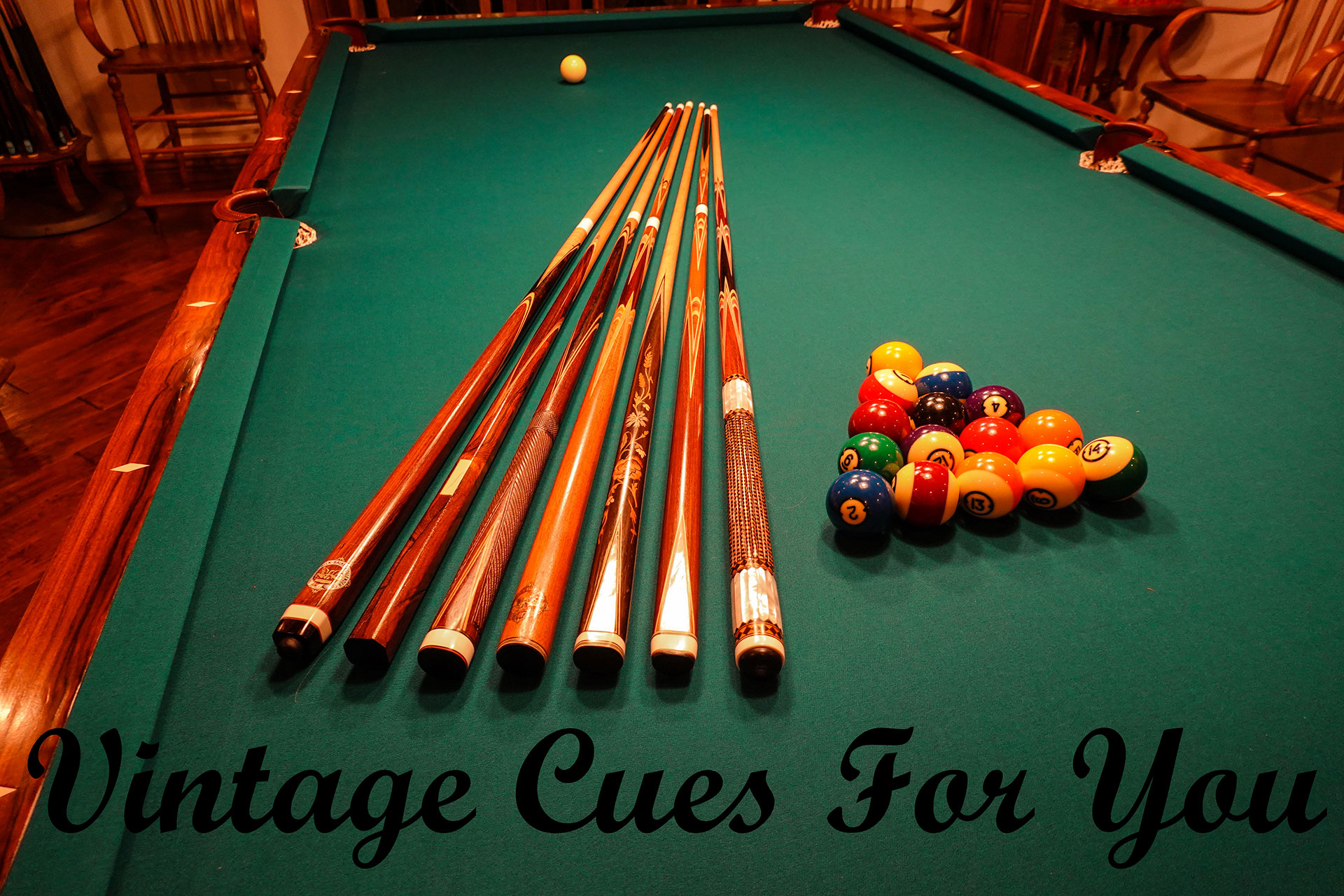The image is a color photograph taken from an angled top-down perspective, showcasing a beautifully maintained pool table with a green felt playing surface and a rich brown wooden rim. The table narrows towards the back and rests on a hardwood floor, with a couple of wooden chairs on either side, contributing to the room’s cozy, vintage ambiance. The table features seven wooden pool cues laid side-by-side, each with different intricate designs, enhancing the overall classic feel. Adjacent to the cues, there is a racked set of old billiard balls, carefully arranged in a triangular formation. The white cue ball is positioned at the very top of the table. Additionally, a few pieces of chalk are visible near the setup. Across the bottom of the photograph, written in thick black cursive script, are the words "Vintage Cues for You," adding a stylish touch to the composition.